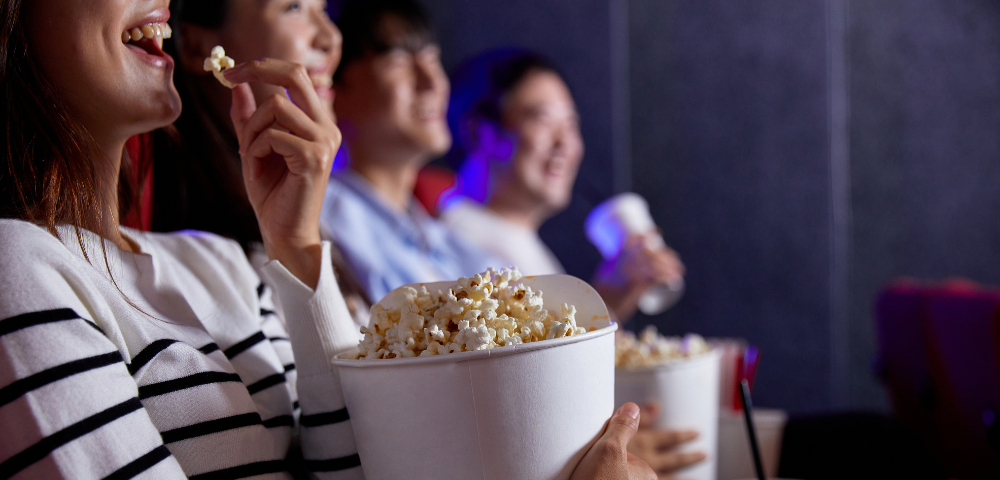This photograph captures the joyful atmosphere of a movie theater, featuring four Asian women clearly enjoying themselves. Seated in plush, bright red velvet chairs against a dark purple theater wall, they are all laughing, indicating a funny moment in the film. The image prominently features a woman in the foreground, dressed in a white and black striped shirt, holding a large white container of popcorn in her lap. To her left, another woman, also laughing, is slightly out of focus but still visible, enjoying the same snack. Farther in the background, two more women are seen, one of whom is holding a white cup with a straw, although they appear more blurry and out of focus. The picture, which is wider than it is tall, cuts off the top half of the face of the woman in the foreground, enhancing the emphasis on the group’s shared laughter and overall enjoyment of the movie experience.